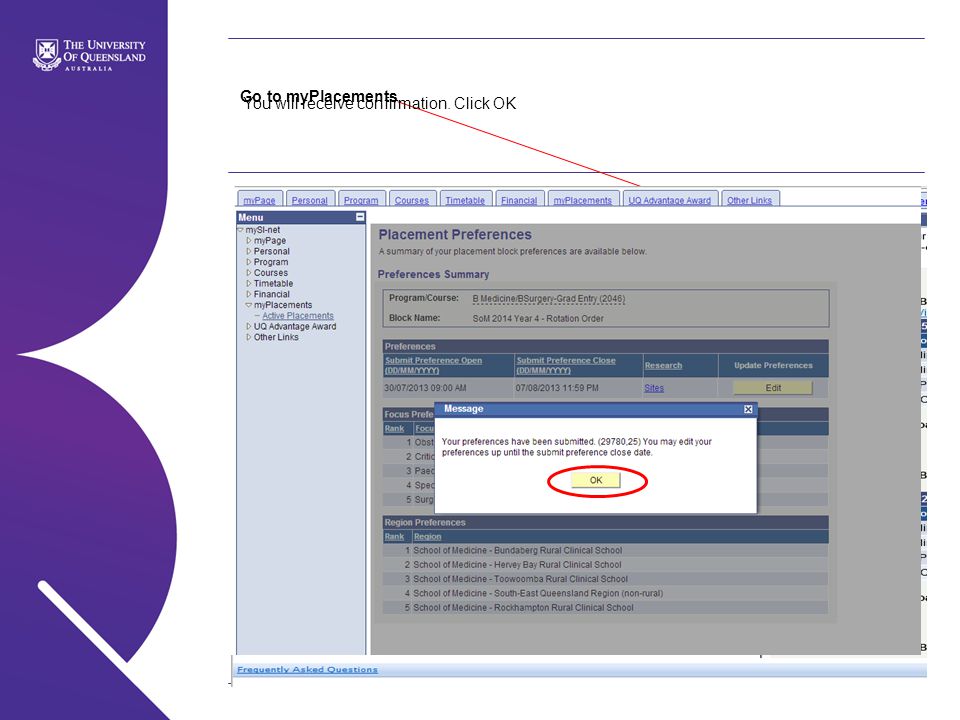This horizontal rectangular image features various elements related to the University of Queensland's student portal. 

On the left side, there is a section with white text on a purple background that reads "The University of Queensland" and beneath that, "Australia." Adjacent to this text is the University of Queensland's logo, which consists of a purple design along the left border of the image.

The top center of the image displays the text "Go to My Placements" in black font. Directly beneath this heading, a thin red line touches one of the menu options on the webpage. The highlighted menu option appears to be labeled "UQ Advantage Award" or something similar.

A horizontal navigation menu spans the top of the image, featuring several items: M Page, Personal, Program, Courses, Timetable, Financial, M Placements, UQ Advantage Award, and other links. An identical vertical navigation menu runs down the left side of the image, containing the same options.

The central area of the image is darkened but still visible. At the top of this section, the heading "Placement Preferences" can be discerned, followed by the text "The summary of your placement block preferences is available below." Below this heading, a section titled "Preferences Summary" lists programs, courses, and block names.

Further down, another section labeled "Preferences" includes a prominent blue button that reads "Student Submit Preference."

Near the middle of the page, a white pop-up message appears on a blue background with white font. The message states: "Your preferences have been submitted. You may edit your preferences up until the submit preference close date." At the bottom of the pop-up, there's an "OK" button set in a horizontal yellow area with a red oval highlighting it horizontally.